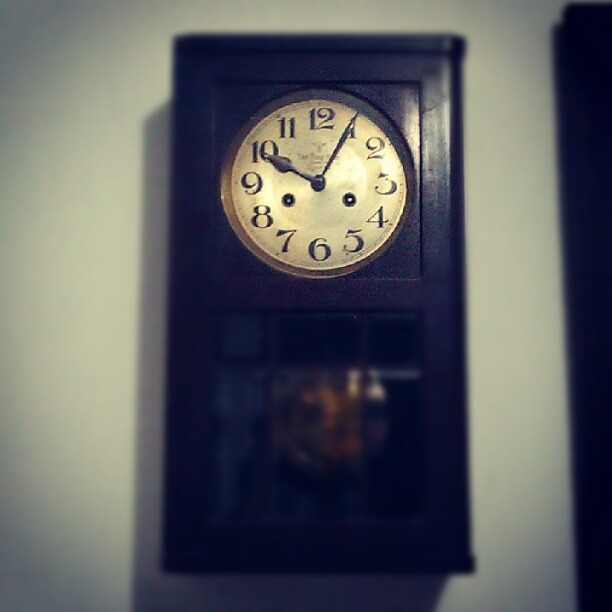In this photograph, an antique pendulum clock is prominently displayed on a green wall. The clock is encased in a tall, upright rectangular frame made of very dark wood that appears almost black or deep brown. The face of the clock is round, colored in a gold or ivory hue, and features black Arabic numerals. The clock hands indicate that it is five minutes past ten. Below the clock face, a small window reveals the clock's pendulum and internal mechanics. The clock casting a shadow on the wall adds to the depth of the image. The photograph has a cool-tone filter with vignette effects, causing the corners to darken and the center to appear lighter. This creates a soft focus on everything except the clock face, emphasizing its details and adding an air of vintage elegance. On the right-hand side, an indistinct dark object, possibly a cabinet, is visible but blurred. The overall composition enhances the antique aesthetic of the clock while leaving some elements intriguingly obscure.